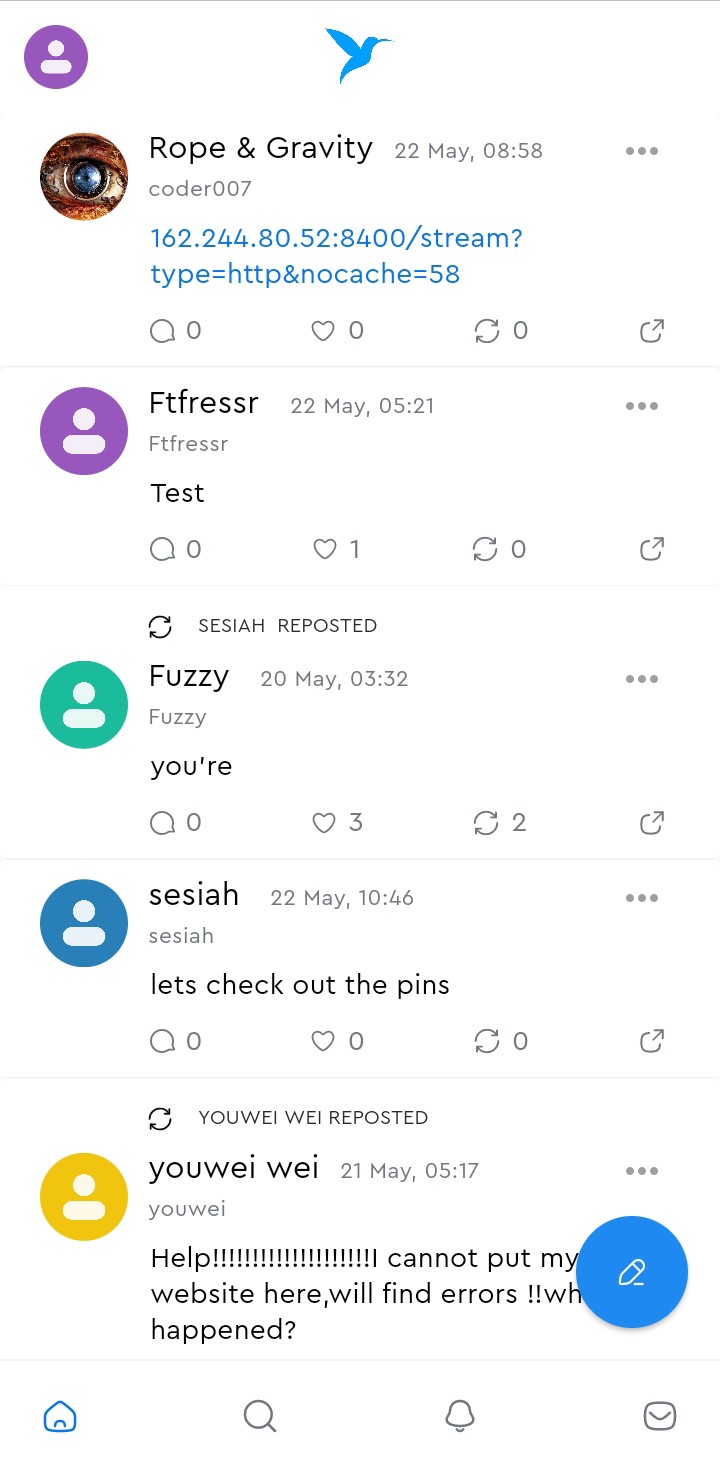This image is a screenshot captured from someone's phone screen. At the top, there is an icon of an eyeball within a profile circle, next to text that reads "rope and gravity." Below this, there is a series of blue-colored numbers resembling a clickable link. Scrolling further down, the text "FTFresser" followed by the word "test" appears.

In the subsequent layer, the word "fuzzy" is displayed, coupled with a grammatical error where "you're" is written as "Y-O-U, apostrophe, R-E." Moving down, a blue circle featuring a person icon contains the text, "let's check out the pins."

At the bottom of the page, there is a yellow person icon next to jumbled text that reads "you wei wei," followed by a plea highlighted with numerous exclamation points, "help!" Accompanied by the declaration, "I cannot put my website here, will find errors," ending with the question, "what happened?" Finally, the screenshot features a blue circle with a pencil icon situated at the bottom.